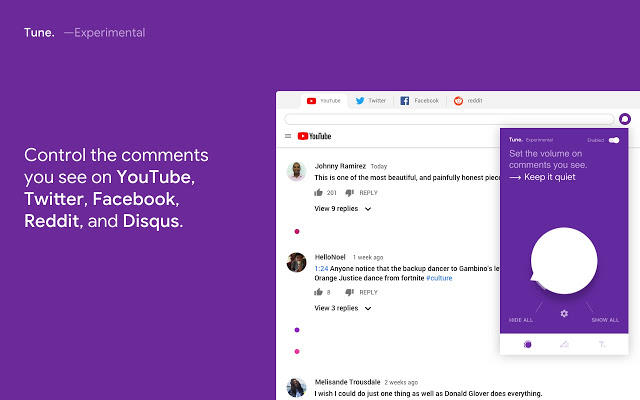The image presents a user interface for a platform designed to control and filter comments across various social media sites. The interface is predominantly purple and features a white box at the top left with the text, "Tune." Next to it, there's a dash followed by the word "experimental." Below this header, a description reads, "Control the comments you see on YouTube, Twitter, Facebook, Reddit, and Disqus."

To the right, a web page mockup is displayed, showing various tabs for YouTube, Twitter, Facebook, and Reddit, with the YouTube tab currently selected. The YouTube interface reveals a series of user comments. The top comment, from Johnny Ramirez, includes a profile picture and reads, "This is one of the most beautiful and painfully honest pieces," but the comment is partially obscured.

Adjacent to the comment section, there is a purple rectangular box containing options to adjust the visibility of comments, labeled "Set the volume on comments you see." Beneath this, a white speech bubble offers the choices "Hide All" and "Show All." Other visible comments include one from a user named "hello Noel," mentioning a backup dancer's move related to Gambino and Fortnite's "Orange Justice" dance. This comment too is truncated. Below it, another partially obscured comment is visible.